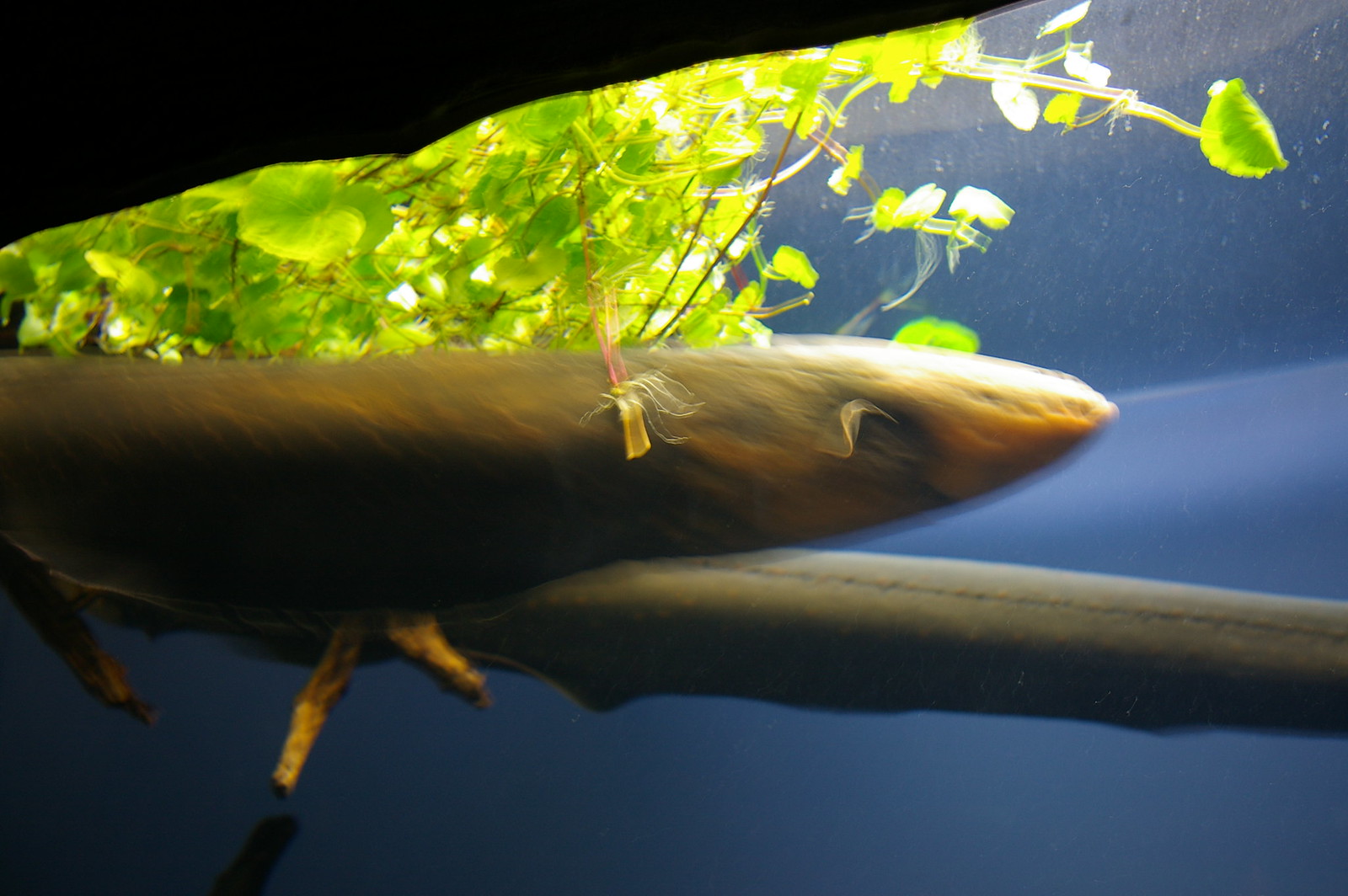This detailed image reveals the underwater scene of an aquarium, likely taken swiftly from an outside perspective, possibly in a zoo. Dominating the frame, a fast-moving fish appears blurry as it swims through the clear water, showcasing its brownish hues and black eye against a dark backdrop. Near the fish, a log or stick-like object, dark brown in color, stretches horizontally and features delicate stems protruding from it. Above this, light-green plants float gracefully on the water's surface, their vibrant colors contrasting with the remnants of daylight filtering through the tank's top. Scattered bubbles enhance the atmosphere, encapsulating the dynamic and vivid aquatic environment.